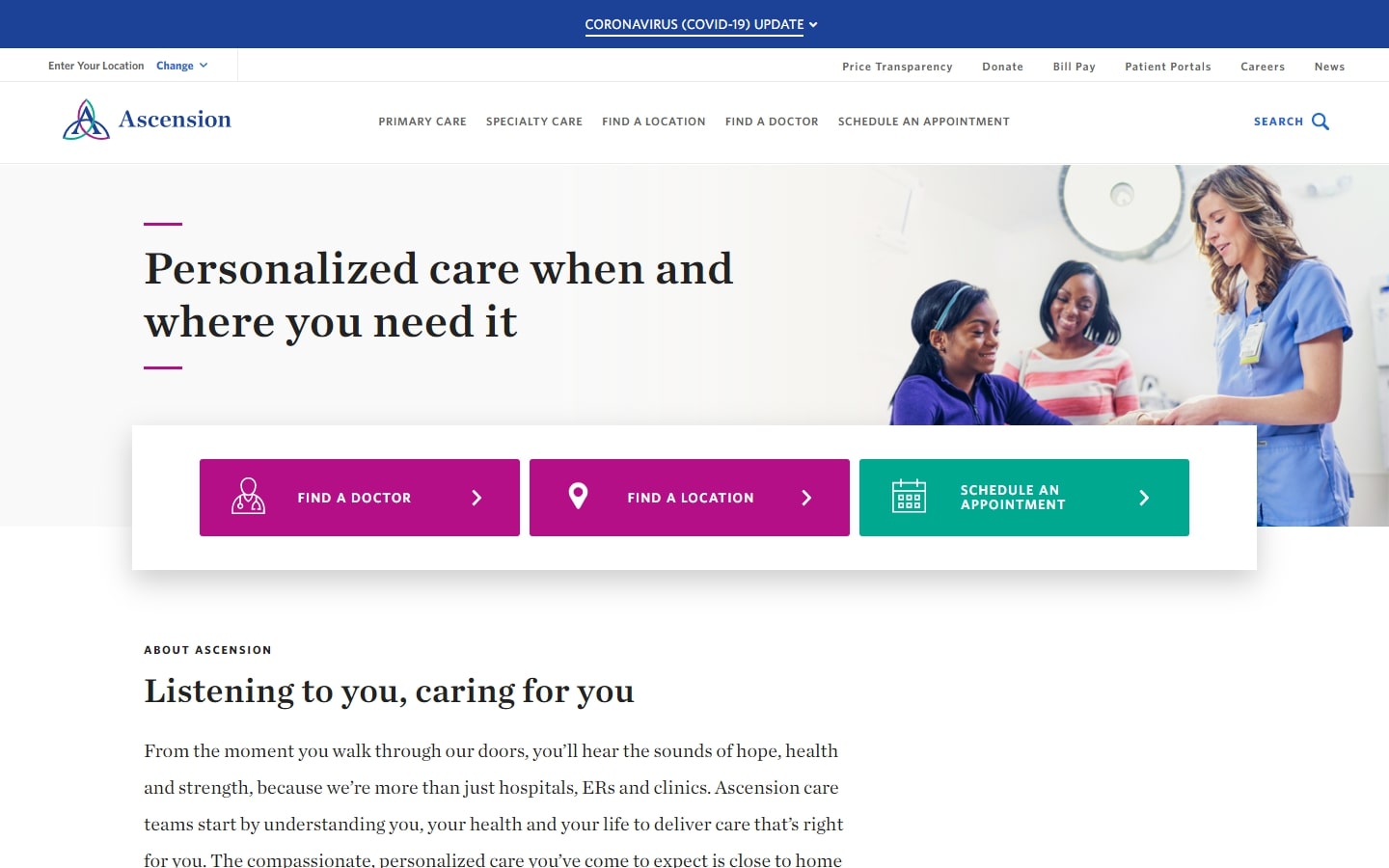The image is a detailed website interface for "Ascension," showcasing various healthcare options. At the top, there is a dark blue background spanning the width of the image, with six small categories aligned underneath. Directly below this area, set against a light gray background, the headline reads "Personalized care, when and where you need it." To the right of the website's title "Ascension," there are five primary categories: "Primary Care," "Specialty Care," "Find a Location," "Find a Doctor," and "Schedule an Appointment," accompanied by a prominent blue search button to their right.

The central part of the image features a nurse in a blue shirt with long hair, assisting two people situated to her left. One individual is wearing a dark blue shirt, while the other sports a pink and white striped shirt and is smiling. Below this scene, three brightly colored rectangles present quick-access options: "Find a Doctor" in purple on the left, "Find a Location" in purple in the center, and "Schedule an Appointment" in green on the right, the latter also featuring a small calendar icon.

At the bottom of the image is a white section titled "About Ascension," with the subtitle "Listening to you, caring for you." This area contains several sentences of small black text explaining Ascension’s mission, located on the left side. The right side of this bottom section remains empty, maintaining a clean and balanced design.